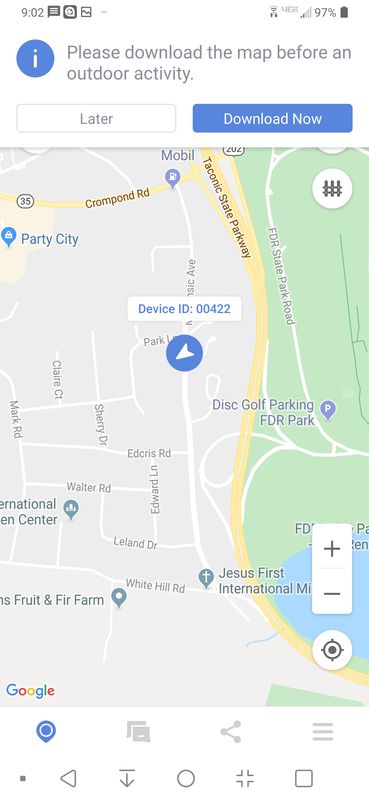This image is a screenshot of the Google Maps app. At the top of the screen, a white alert banner features a blue eye icon on the far left. To the right of the icon, small gray text reads, "Please download the map before an outdoor activity." Below this alert, on the left side, a large box labeled "Later" can be seen, and to its right, another large box labeled "Download Now" is present.

Dominating the screen is the map itself. Centrally placed on the map is a blue circular icon with an arrow, accompanied by a white rectangle displaying the device ID. On the bottom right of this central area, plus and minus icons in boxes allow zooming in and out, while below them is a round location reset icon.

At the bottom of the screen, multiple function icons are visible. From left to right, there is a location pin drop icon, a Windows icon, a share icon, and a menu icon. Further below, the bottom-most row displays a small gray dot in the right corner, followed by a triangular play button oriented to the left, a download icon, a home screen icon, an adjust view icon, and finally, a square box icon.

This detailed layout captures the intricacies of the Google Maps interface, highlighting both navigational aids and functional icons.